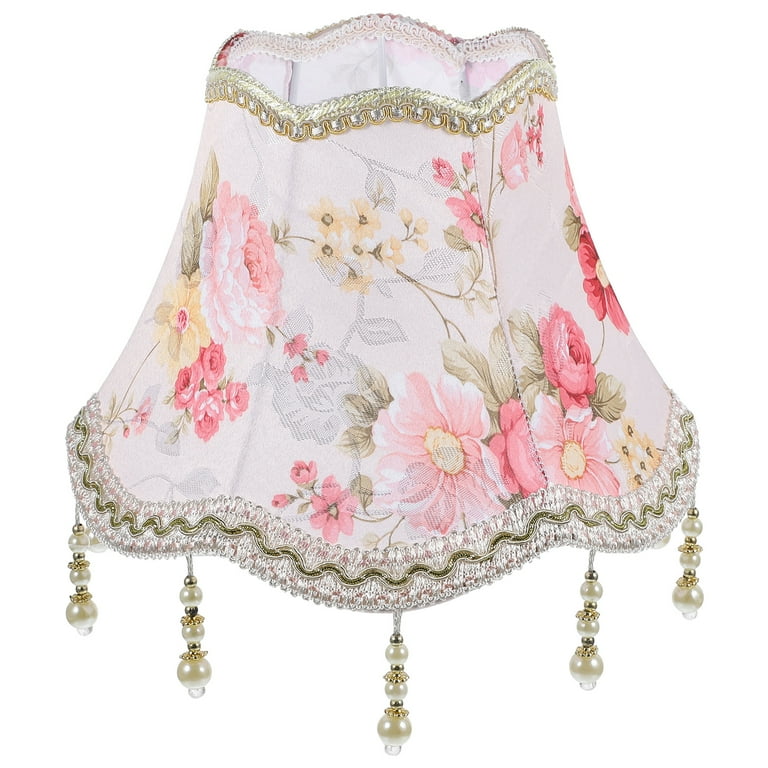The image features a premium, luxurious lampshade positioned centrally and extending from the top to the bottom of the frame. The lampshade boasts an ornate, intricate design reminiscent of Japanese aesthetics, with a beautiful, very light purple background adorned with a rich variety of flowers, including chrysanthemums, roses, zinnias, yellow daffodils, and other floral motifs. The flowers showcase a spectrum of colors such as pink, red, yellowish-orange, and are complemented by dark green leaves. The lampshade is further embellished with delicate, pearl-like tassels, five of which are visible and likely encircle the entire base. These tassels dangle from a fancy, embroidered edging, enhancing its opulent and elegant appearance. The overall effect is one of beauty and luxury, suggesting a setting fit for someone rich or of royal standing.